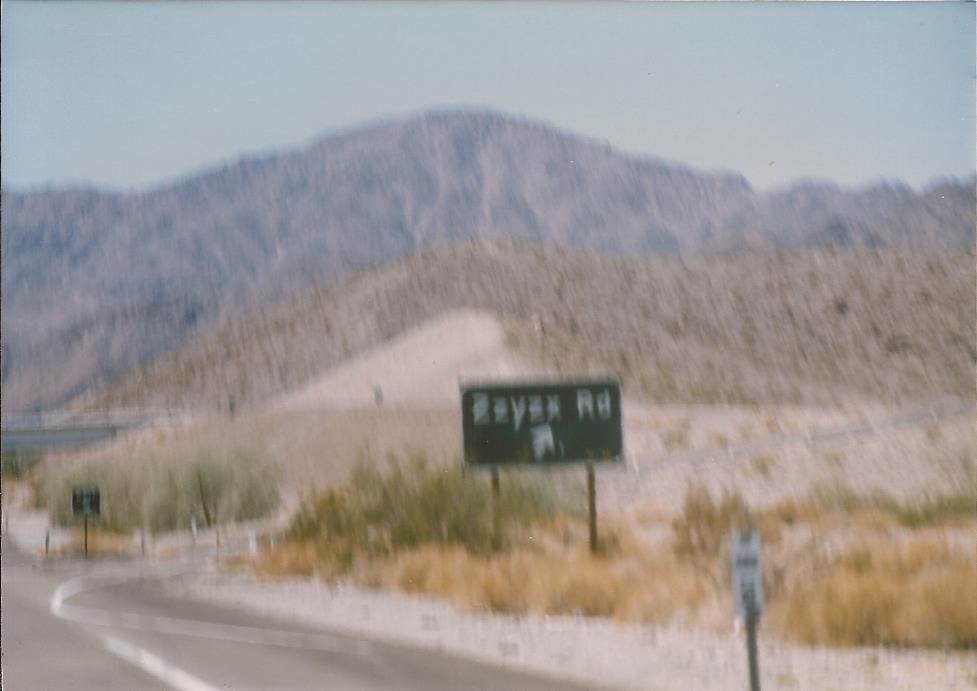In this somewhat blurry image, the sky is a delicate shade of light blue, creating a serene backdrop. Below the sky, a series of lush, green mountains covered densely in trees dominate the scene, providing a striking contrast to the adjacent hills, which are marked by patches of brown and sandy hues. The foreground is characterized by a mix of tall grasses and weeds, presenting a spectrum of browns interspersed with hints of green. A highway cuts through the landscape, leading the eye toward a notable black sign visible in the background. In the vicinity, a white fence with distinct posts adds an element of structure. Additionally, a smaller white sign with black text is present, alongside a prominent sign displaying "Bayer Road" with a clear directional arrow pointing to the right.